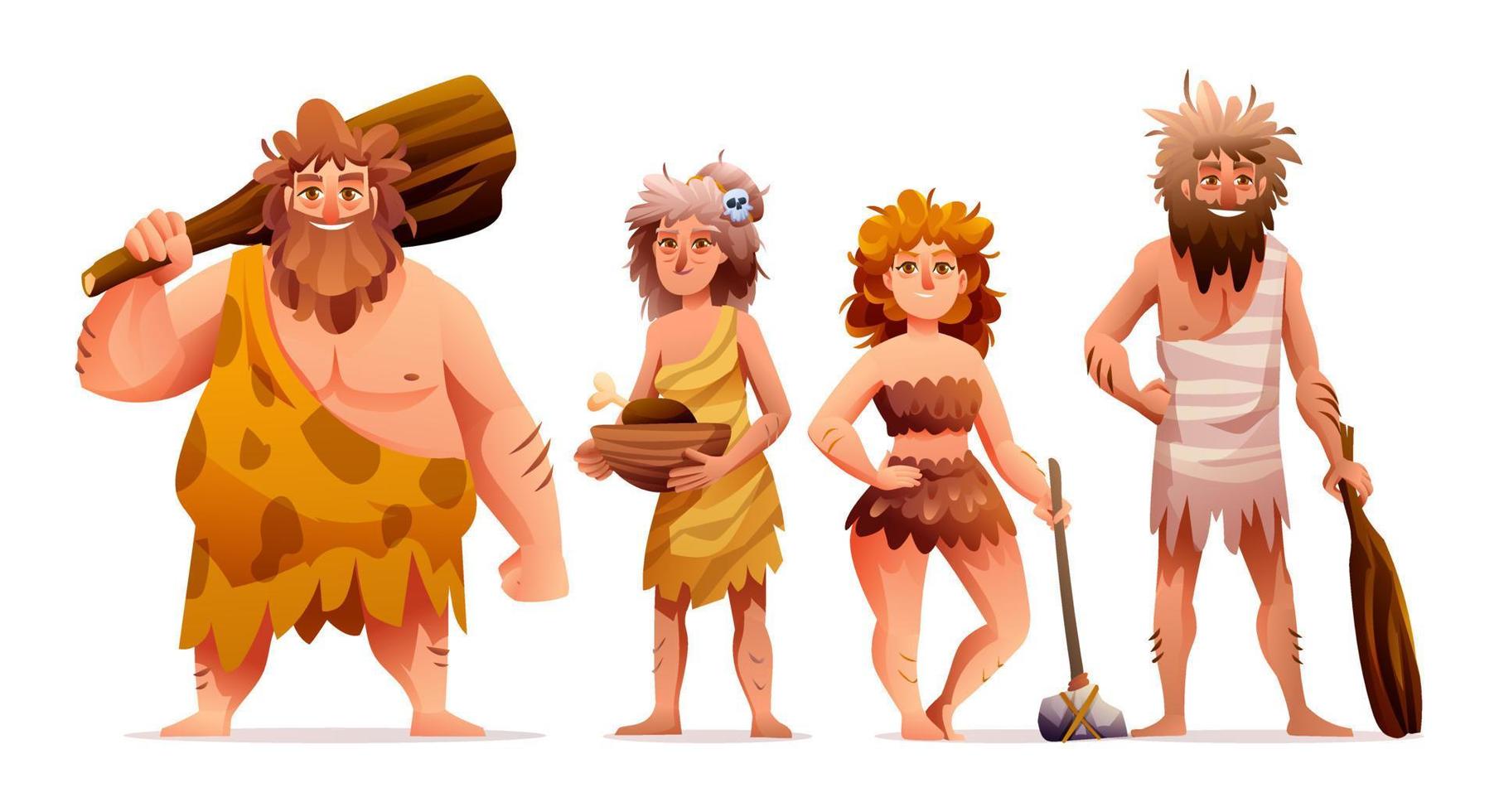The image depicts four animated characters resembling a modern reinterpretation of the Flintstones, all standing side by side and smiling in a computer-generated graphic. On the far left is a stout, heavy-set man dressed in a cheetah skin tunic that drapes over one shoulder, leaving the other shoulder bare, and functions as a skirt at the bottom. He has disheveled long brown hair, a thick mustache, and a matching beard, and holds a large wooden club resting on his shoulder. Next to him is an older woman, identified by her shaggy gray and brown hair tied back with a skull pin. She is dressed in a one-shoulder yellow and gold dress and holds a bowl half of a coconut containing a drumstick. The third character is a younger, full-bodied woman with curly shaggy brown hair, clad in a brown two-piece outfit that includes a tube top and a short skirt. She wields a primitive-looking hammer or stone mallet in her hand. Finally, on the right stands the tallest character, a lean man with long shaggy brown hair, a thick mustache, and beard. He wears a tunic with white and gray stripes over one shoulder, extending into a skirt at the bottom, and holds a smaller wooden club. Overall, the characters evoke a whimsical, prehistoric atmosphere reminiscent of a Flintstones-like environment.